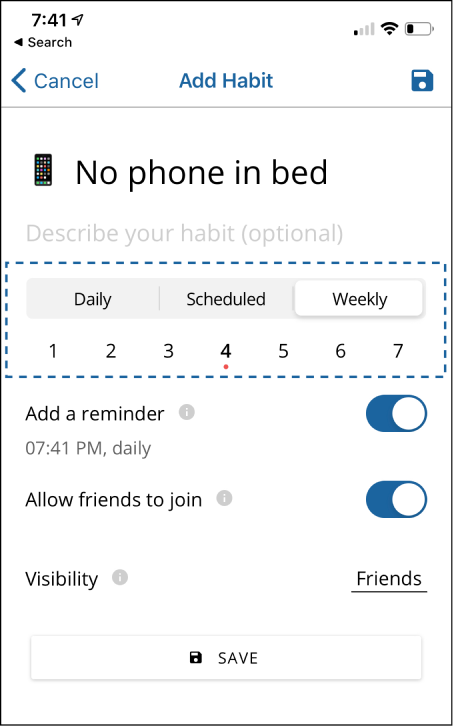A feature-rich alarm-based app is displayed on a phone screen at 7:41 PM, signified by the time at the top. The status bar also shows minimal battery, a single Wi-Fi signal, and a network bar on the right. The primary interface centers around habit management, indicated by the 'Add Habit' option at the bottom.

On the left side, a 'Cancel' option with an arrow is visible, while the right side features a floppy disk save icon for saving preferences. In the main section, a habit named 'No phone in bed' is input, with a gray placeholder reading 'Describe your habit (optional)' beneath it. 

Scheduling options are displayed, with the 'Weekly' setting active. Numbers 1 through 7 indicate the days of the week, with a red dot under the number 4, likely denoting a specific selection. 

A prompt to 'Add a reminder' includes a white button, and below that, a time setting shows 7:41 PM daily. Additionally, there's an option to allow friends to join the habit, with visibility settings set to 'Friends'. 

At the bottom of the screen, a prominent 'Save' button allows the user to finalize their settings.